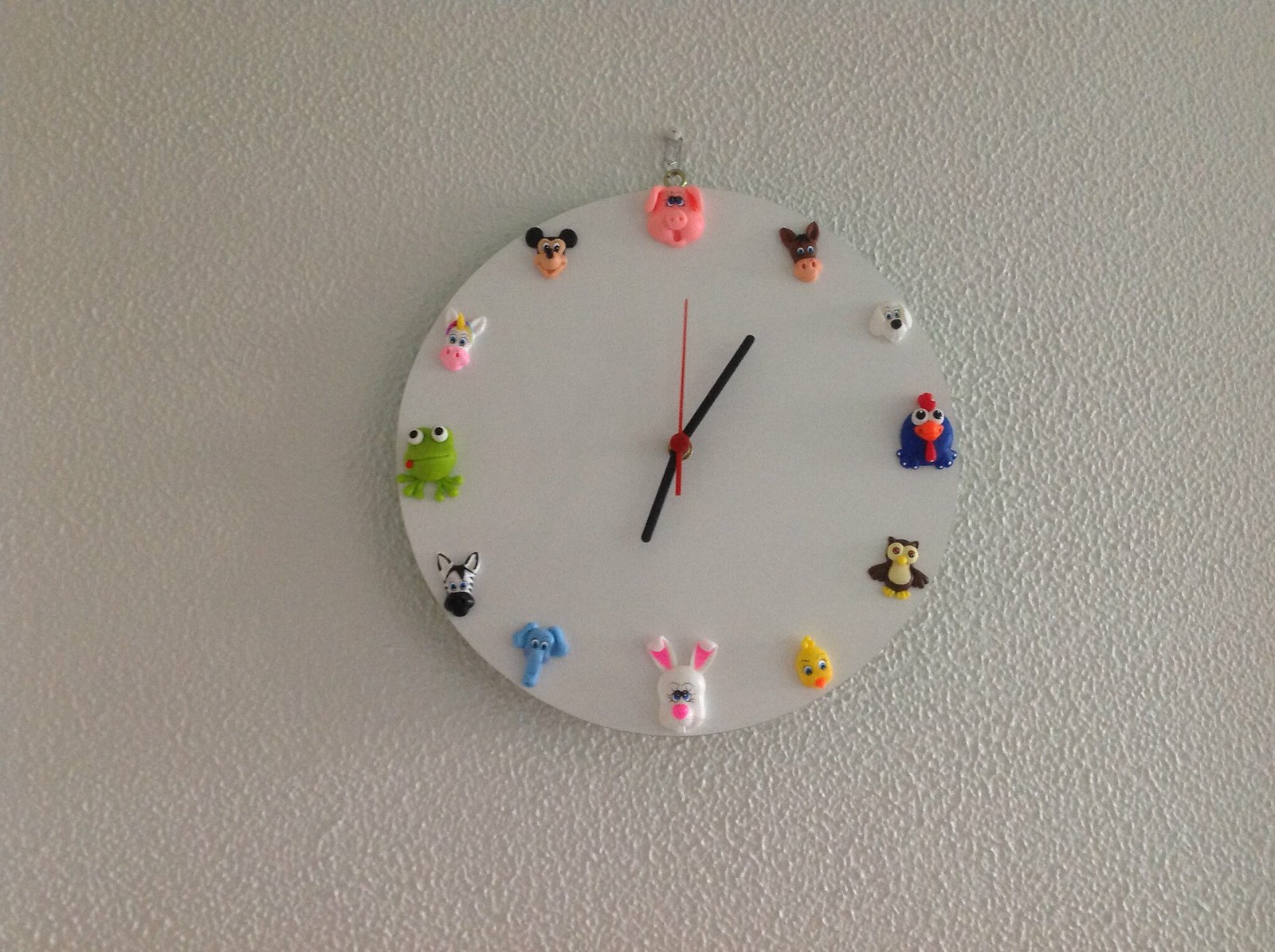The image depicts a uniquely styled circular wall clock featuring a frosted glass face. Unlike traditional clocks with numerical hour markers, this clock showcases a variety of animal faces in place of numbers. The clock is equipped with an hour, minute, and second hand. The animals depicted include a pig, horse, dog, rooster, owl, duck, rabbit, elephant, zebra, frog, donkey or cow, and a mouse. The arrangement of these animal faces does not seem to follow any logical order, adding an eclectic and whimsical touch to the design. The clock combines functionality with a playful aesthetic, making it a distinctive decorative piece.